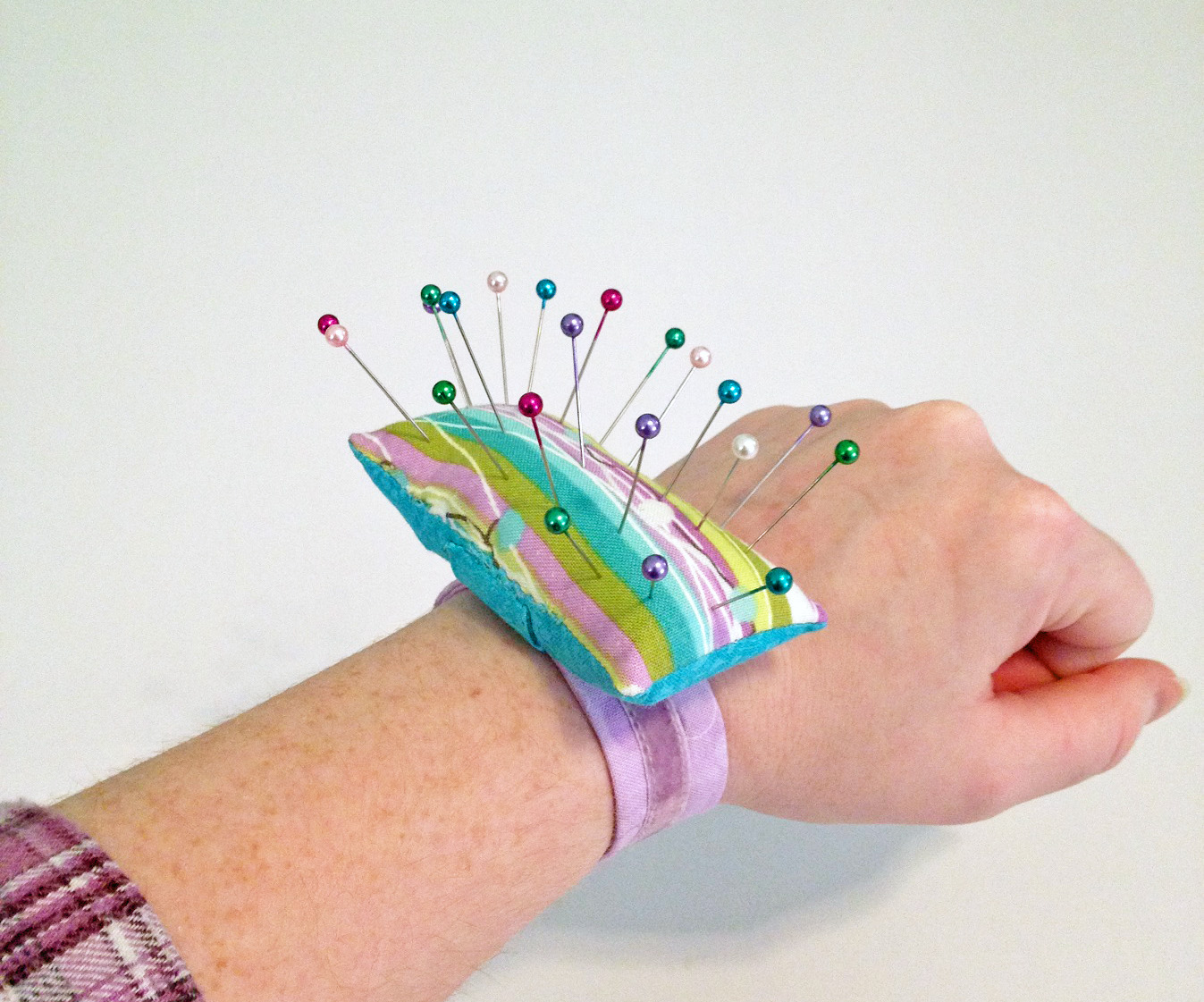A close-up image features the left arm and hand of a freckled person, likely a woman, based on the length of their nails. Their hand is clenched into a fist, highlighting a handmade pin cushion strapped around their wrist with a pink velcro band. The pin cushion itself is an intricately designed padded rectangle, combining hues of blue, green, purple, pink, and white. Various colored pins, with pearlized tips in shades of blue, green, silver, purple, and red, protrude from the cushion. The person is dressed in a maroon plaid shirt, and the background is a neutral gray, creating a clean and focused composition that accentuates the details. This visually harmonious scene suggests a crafting or sewing activity, emphasizing the practicality and neat organization of the colorful pins in the pin cushion.